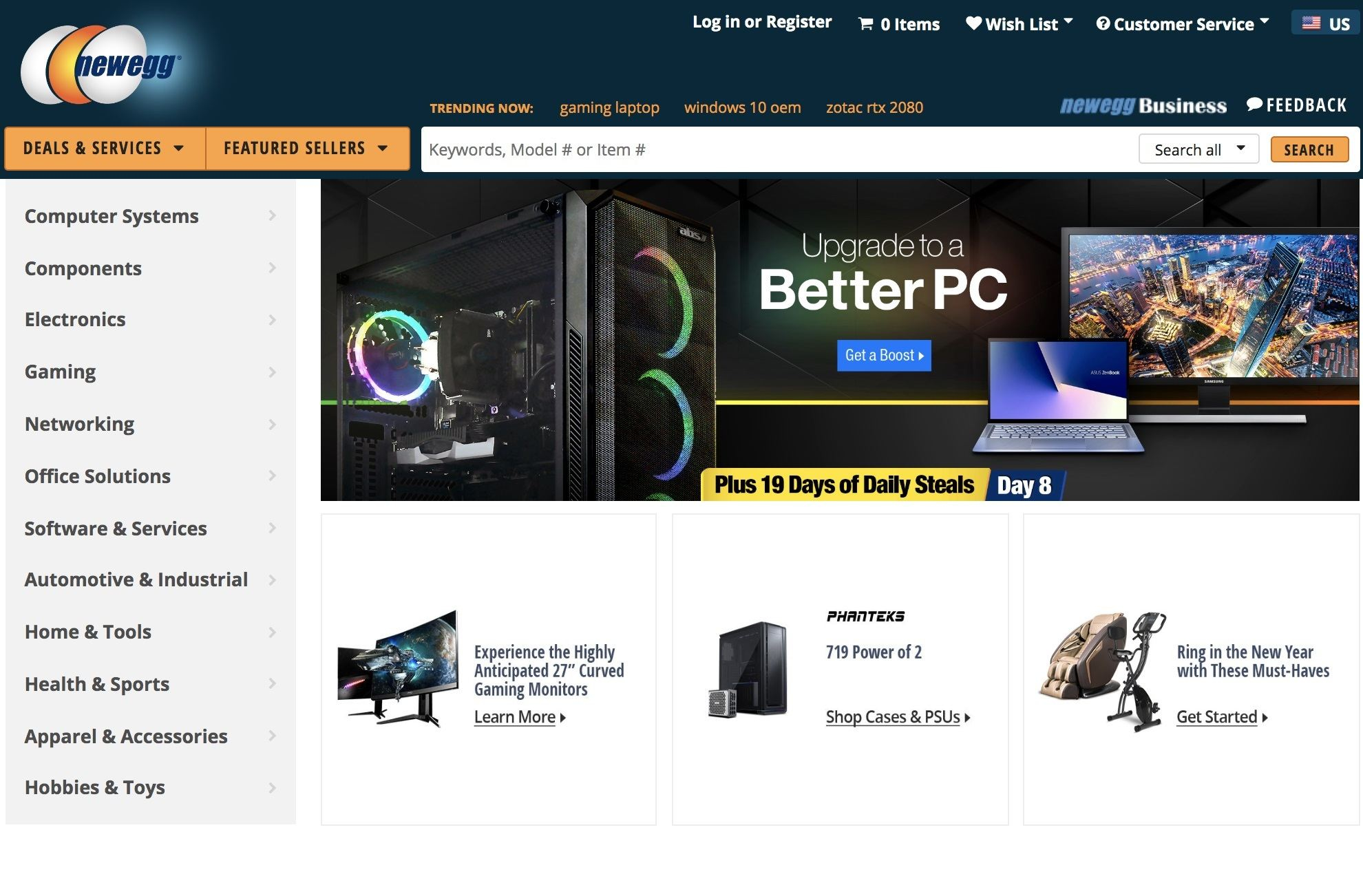The top of the image features an icon on the left with two white eggs and one golden egg. Adjacent to this icon, "New Egg" is written, followed by options to the right that include "Login," "Register," and counters for items in the wish list, customer service, and additional user-based categories. Below these, there are trending sections like "Gaming Laptop," "Windows 10," "Zotac RTX 2080," "New Egg Business," and "Feedback."

Two orange buttons with drop-down tabs labeled "Deals & Services" and "Featured Sellers" appear prominently, alongside a search box to the right where users can enter keywords, model numbers, or item numbers. Beneath this section, the main image displays a computer setup with a TV or computer monitor and a laptop, accompanied by the tagline "Upgrade to a Better PC" and a blue button labeled "Get a Boost."

Additionally, it advertises "19 Days of Daily Steals - Day 8," and a banner promoting "Experience the highly anticipated 27-inch curved gaming monitors," with a "Learn More" button for more details. On the right side, the phrase "A 719: Power of 2" is mentioned, encouraging users to "Shop Cases and PSUs."